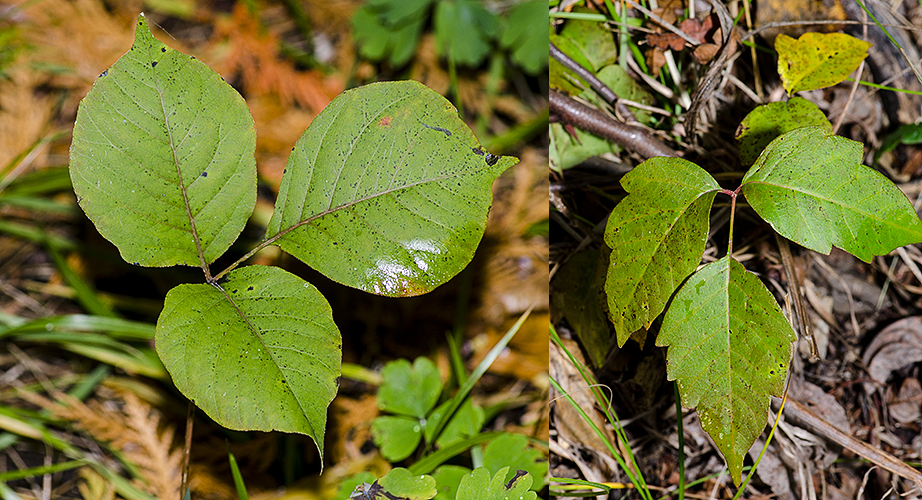The image consists of two side-by-side pictures, each showcasing a distinct plant with three leaves. Both plants are set against a ground covered in a mix of dead leaves, pine needles, clovers, and other forest debris typical of a natural, wilderness environment.

On the left side, the plant features three fairly large, oval or round leaves, appearing healthy despite the presence of some black spots which may be natural to the plant. The leaves are symmetrical and rounded, set against a ground that is predominantly green with some brown areas. Below these leaves, various dried leaves, pine needles, and clovers can be observed.

The right side of the image displays another plant, also with three leaves, but these are more triangular in shape with slight points and rough edges, and a hint of pink on the stem. The ground beneath this plant looks more dead and brown, indicating a later season with more decomposed material. The leaves here also have black spots and appear more drooped and asymmetrical compared to the ones on the left. 

The side-by-side comparison might be illustrating the differences between similar-looking plants, potentially highlighting distinctions between poison ivy and other tri-leaf plants.